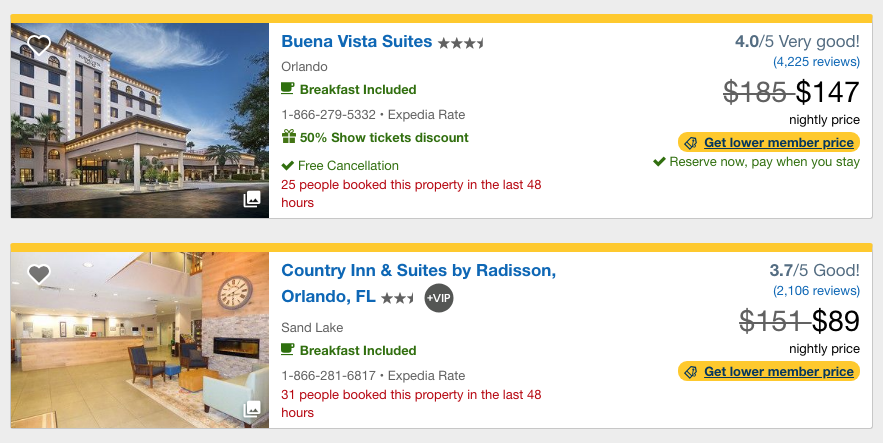The image is a detailed screenshot comparing two different hotel results for accommodations in Orlando, Florida. 

**Left Side - Buena Vista Suite, Orlando:**
- Hotel Name: Buena Vista Suite
- Location: Orlando
- Amenities: Breakfast included
- Contact Information: Phone number provided
- Discount Details: Expedia rate, 50% off, show tickets discount
- Cancellation Policy: Free cancellation
- Rating: Not specified, but mentioned as "very good"
- Price: $147 per night
- Additional Offers: Get a lower member price, reserve now and pay when you stay
- Visual: Thumbnail picture of the hotel exterior
- Reviews: 4,227 reviews

**Right Side - Country Inn and Suites by Radisson, Orlando, Florida:**
- Hotel Name: Country Inn and Suites by Radisson
- Location: Sand Lake, Orlando, Florida
- Amenities: Breakfast included
- Rating: 3.7 out of 5, rated "good"
- Price: $89 per night
- Additional Offers: Get a lower member price
- Visual: Thumbnail picture of the hotel interior
- Reviews: 2,106 reviews

Overall, the right side showcases a more modestly priced option with a slightly lower rating but notable for its considerable number of reviews and interior image. The left side presents a higher-rated, pricier hotel with additional discount features and promising reviews, complemented by an exterior image of the property.